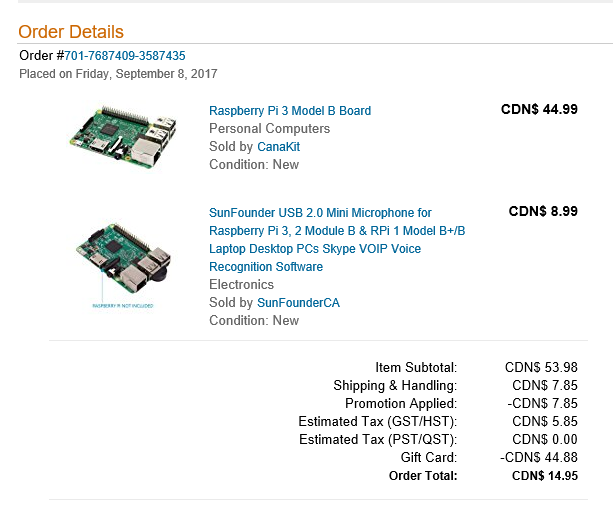Screenshot of Amazon Order Details from September 8, 2017:

The screenshot displays the order details for a purchase made on Amazon, characterized by its distinctive orange and white aesthetic. At the top left, highlighted in orange text, is the label "Order Details." Directly below that is the order number, followed by the placement date, "Friday, September 8th, 2017," in pale gray text.

The items listed in this order include:

1. **Raspberry Pi 3 Model B Board**: This item was purchased for $44.99 CAD. It was sold by CanaKit and listed in new condition.

2. **SunFounder USB 2.0 Mini Microphone**: This accessory is compatible with the Raspberry Pi 3 Model B, Raspberry Pi 1 Model B+, B laptops, desktop PCs, Skype, and voice recognition software.

The detailed view provides a comprehensive look at both the receipt and the specifications of the items bought, ensuring clarity on purchase information and item compatibility.